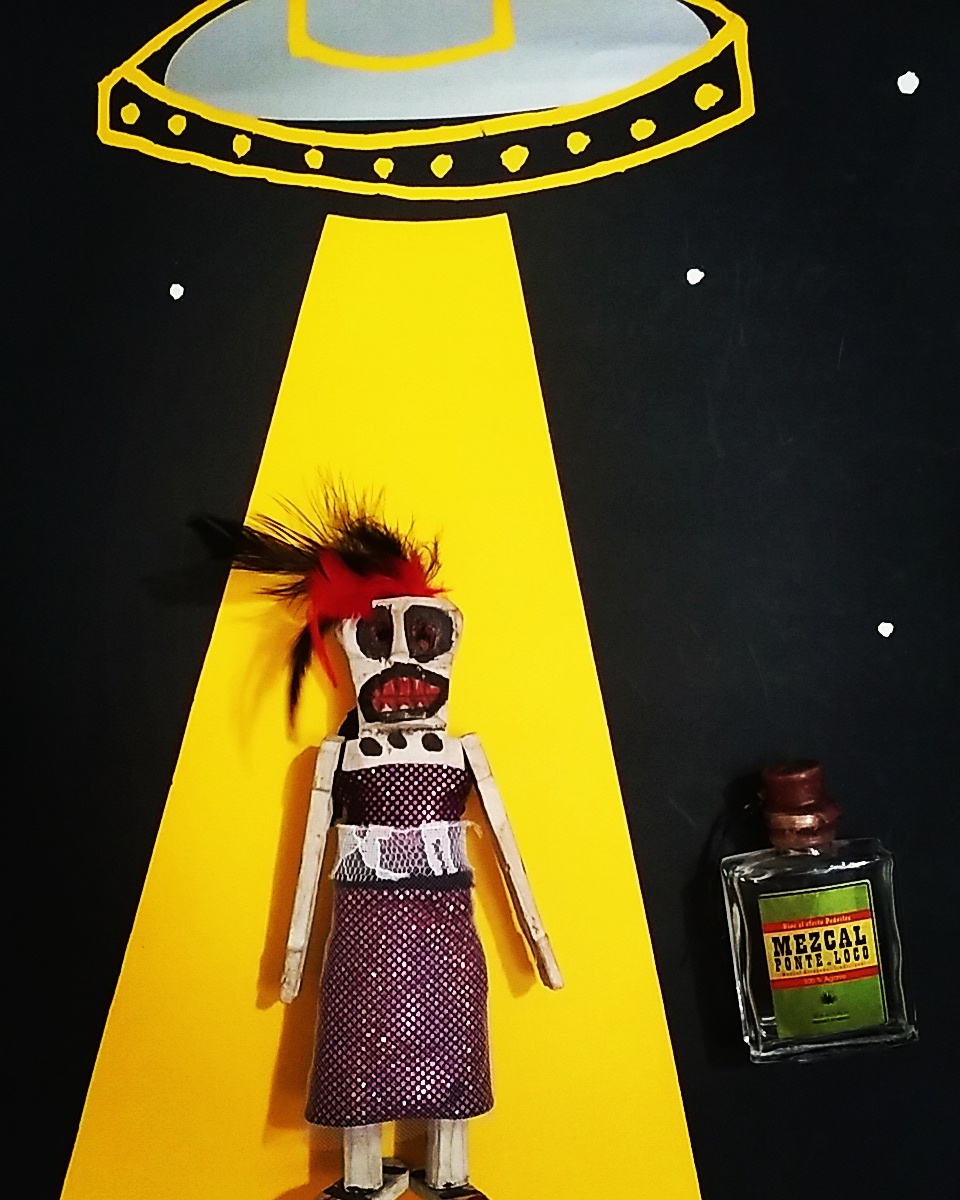The image is an artistic depiction of what appears to be a paper mache-style puppet or doll, characterized by striking features and a dramatic setting. The puppet, which seems to possibly represent a Mexican figure, is designed with a humanoid shape and is adorned in a glimmery dress that suggests sequins but is actually made from paper. It wears a sleeveless blouse tucked into a skirt and boasts vivid red and black feathered hair. The face of the puppet is striking, with wide-open jaws revealing sharp, pointed black teeth and a vibrant red interior. Positioned near the puppet is a small glass bottle, clearly labeled "Mezcal" in green text, likely indicating an alcoholic beverage. Dominating the background is a night sky depicted in solid black with a sprinkling of four white star-like dots. Above the puppet, a gray and yellow spaceship looms, emitting a triangular yellow beam of light that envelops the puppet, suggesting an alien abduction scenario.